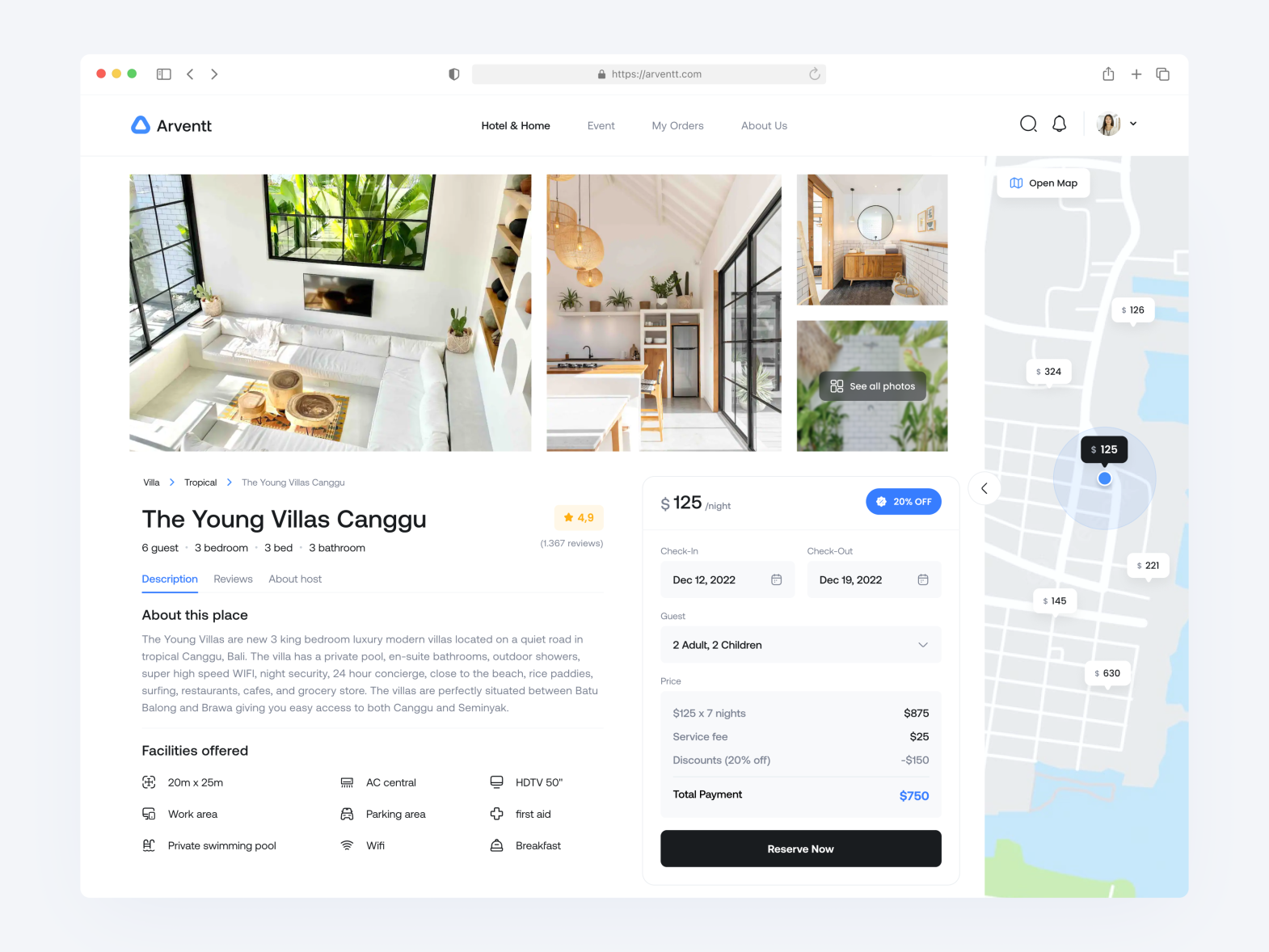This digital image showcases a web interface intended for a housing and event rental website. The website features a structured layout adorned with a gray border surrounding a predominantly white central page. In the upper left-hand corner, a three-circle icon displays small red, yellow, and green circles. Adjacent to this is the URL "https://arvent.com," followed by a blue triangle icon beside the brand name "Arvent."

The top navigation bar contains menu items such as "Hotel and Home," "Event," "My Orders," and "About Us," with a search bar, notifications icon, and profile icon positioned on the right. Below this bar, the main content area includes a map indicating various price points like $126, $324, $125, $145, $221, and $630, alongside embedded images of luxurious housing.

The displayed housing options feature elegant interiors such as a white sectional sofa, a white table complemented by oak chairs, and an oak-finished bathroom with a large mirror and tiled walls. One specific listing, "The Young Villas," is detailed with information including accommodations for 6 guests, 3 bedrooms, and 3 bathrooms. It has a 4.9-star rating and offers pricing at $125 per night with a 20% discount.

Further booking details include:
- Check-in: December 12, 2022
- Check-out: December 19, 2022
- Guests: 2 adults, 2 children.

Cost breakdown:
- Total for 7 nights at $125: $875
- Business fee: $25
- Discount (20% off): -$150
- Total payment: $750

A prominent "Reserve Now" button in black invites immediate action. Additionally, the facility amenities are listed: a 20 x 25 meter area (purpose unspecified), a work area, private swimming pool, central air conditioning, parking area, Wi-Fi, a 50-inch HDTV, first aid, and breakfast provided.

Overall, the image effectively presents a detailed, high-end rental listing with user-friendly navigation and comprehensive booking information.